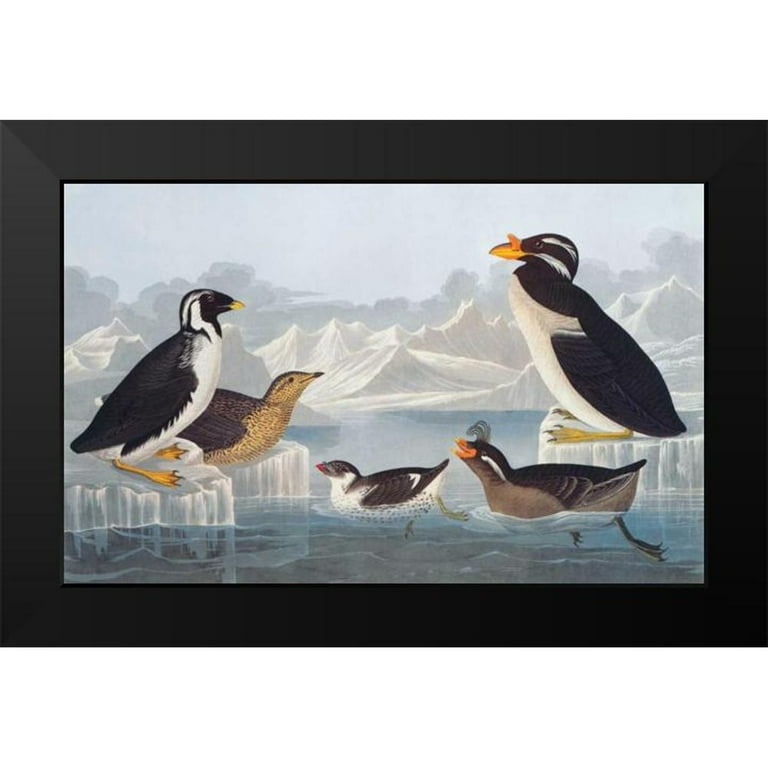The painting, surrounded by a black wooden frame, captures a lively scene of various birds set against a serene daytime backdrop with light blue sky and white glaciers. At the center and right of the painting, five distinctive birds can be seen. The foreground features an elegant black-and-white penguin with yellow feet, standing on the left side and gazing intently to the right. Just below it, in the water, is a bird resembling a duck, characterized by its dark brown back and lighter brown underside, also looking to the right.

In the middle of the water, two birds are swimming—one displaying black-and-white plumage while the other showcases dark brown and white feathers. These two birds, possibly ducks, seem to be floating effortlessly on the varying shades of blue water, with hints of green feathers on one of their heads and an orange beak. Meanwhile, on the far right, another penguin stands firmly on an iceberg. This penguin, sporting a black and white body with an orange beak, appears to be gazing in the opposite direction, leftward.

The painting, with its intricate details and black frame, resembles an ideal piece of art ready to be displayed. The overall scenery, complete with icebergs and glaciers in the background, infuses a sense of cold tranquility, capturing the essence of an arctic landscape teeming with diverse avian life.